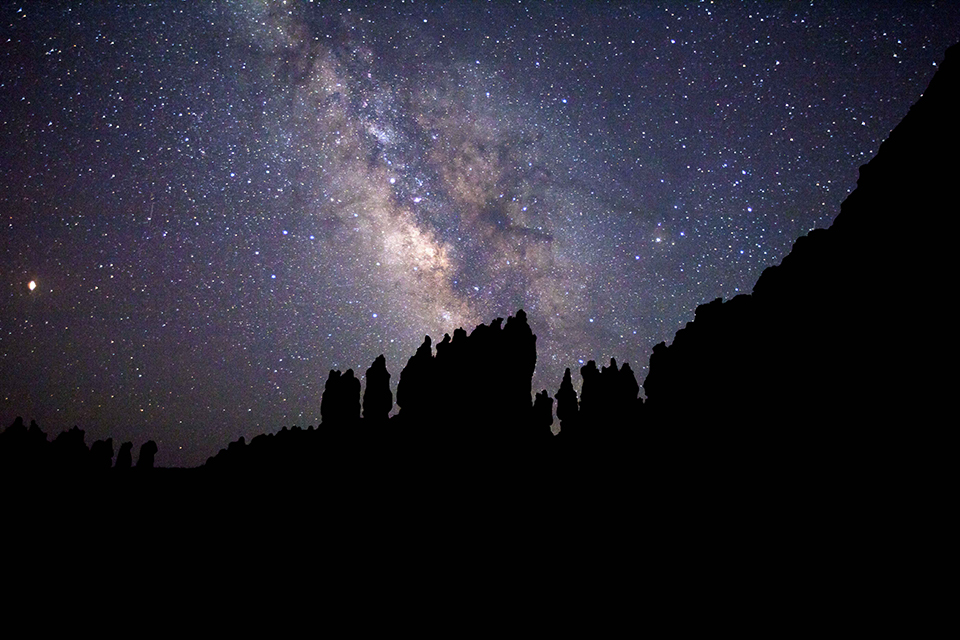This captivating nighttime photograph captures a vast starry sky from a mountaintop perspective. The jagged mountain ridge, silhouetted in black, stretches diagonally from the bottom left corner to the upper right, with a few shadowy trees dotting the base. The true spectacle lies in the night sky beyond, densely packed with countless stars that appear as tiny pinpricks of light. Dominating the center is the Milky Way, a clear formation of our galaxy with intricate patterns of brownish and tan clouds amidst the bright star field. Notably, a single, exceptionally bright star—possibly the North Star—shines prominently on the left side of the image. The photograph is sharp and devoid of any text, perfectly showcasing the majestic interplay of the mountains and the celestial wonders above.